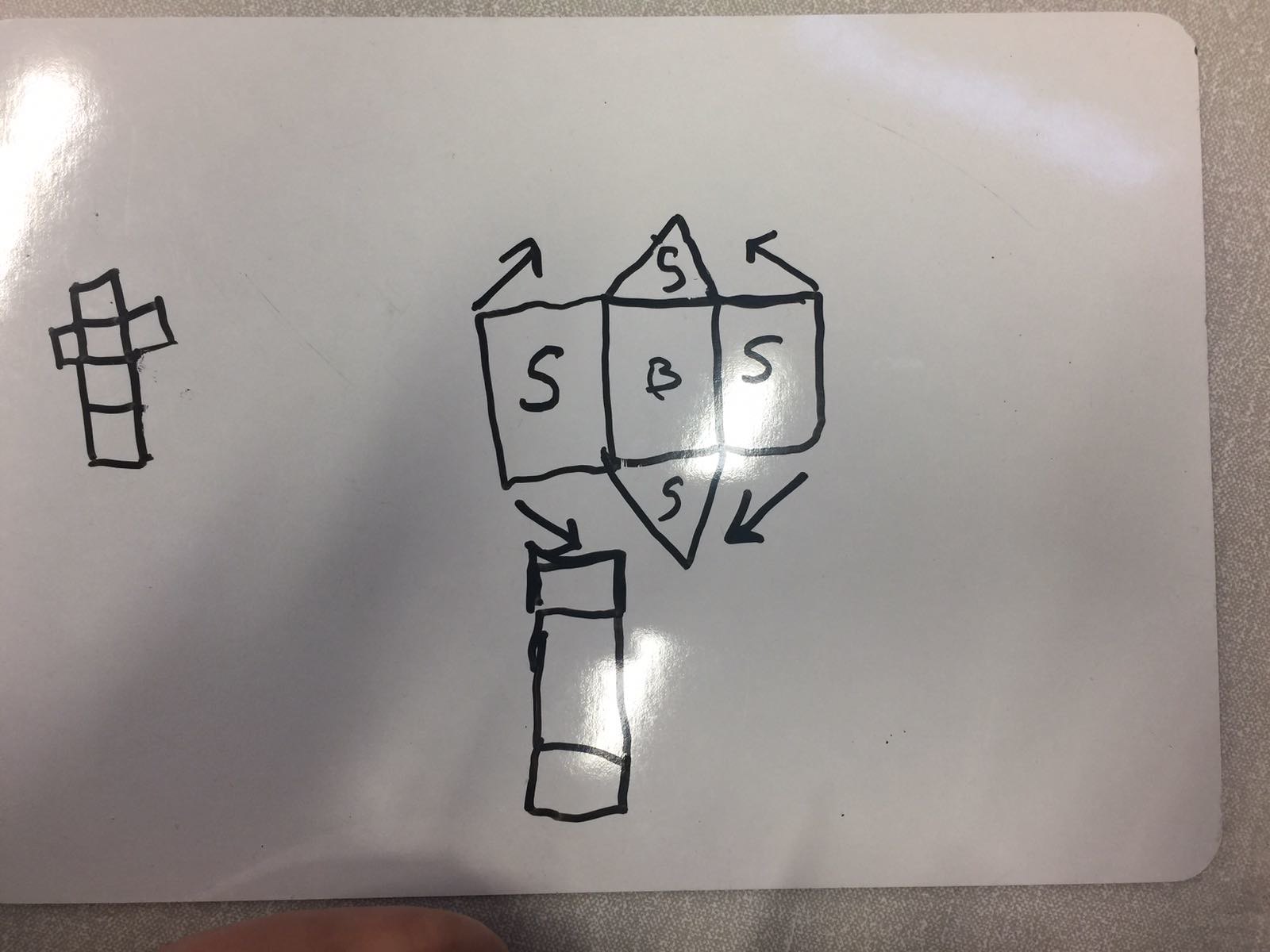A highly detailed magic marker drawing on a white dry erase board, with the following elements:

- An encompassing gray line starts from roughly a quarter-inch from the left edge, runs horizontally to an inch from the right edge, curves around the corner to descend on the right side, and finally curves back about an inch from the bottom to traverse horizontally to the left edge.
  
- The dry erase board's surface is white, with several reflections of light visible. Near the top left corner is a noticeable light reflection. Below this, and slightly to the right, is a cross-shaped figure composed of four vertical squares intersected by three horizontal squares.
  
- To the right of this cross, closer to the center, is another glare of light. A third glare is visible below and to the left of this central glare.
  
- Centered horizontally, three rectangles are aligned from left to right. Above and below the middle rectangle, triangular shapes extend upward and downward, respectively.
  
- Each of the triangles at the corners of the middle rectangle has an arrow pointing inward and upward toward the triangle. The left, right, top, and bottom triangles each contain the letter 'S.'
  
- The first rectangle contains the letter 'S', the middle one an 'N', and the last one an 'S'. Below the middle rectangle's 'S'-bearing triangles, pointing downward from the bottom left, is an arrow resembling a small rectangle with two horizontal lines intersecting it at about one-third intervals.
  
- Finally, at the bottom of the board, about two inches from the left edge, a partial thumbprint can be seen, characterized by its distinct ridge patterns.